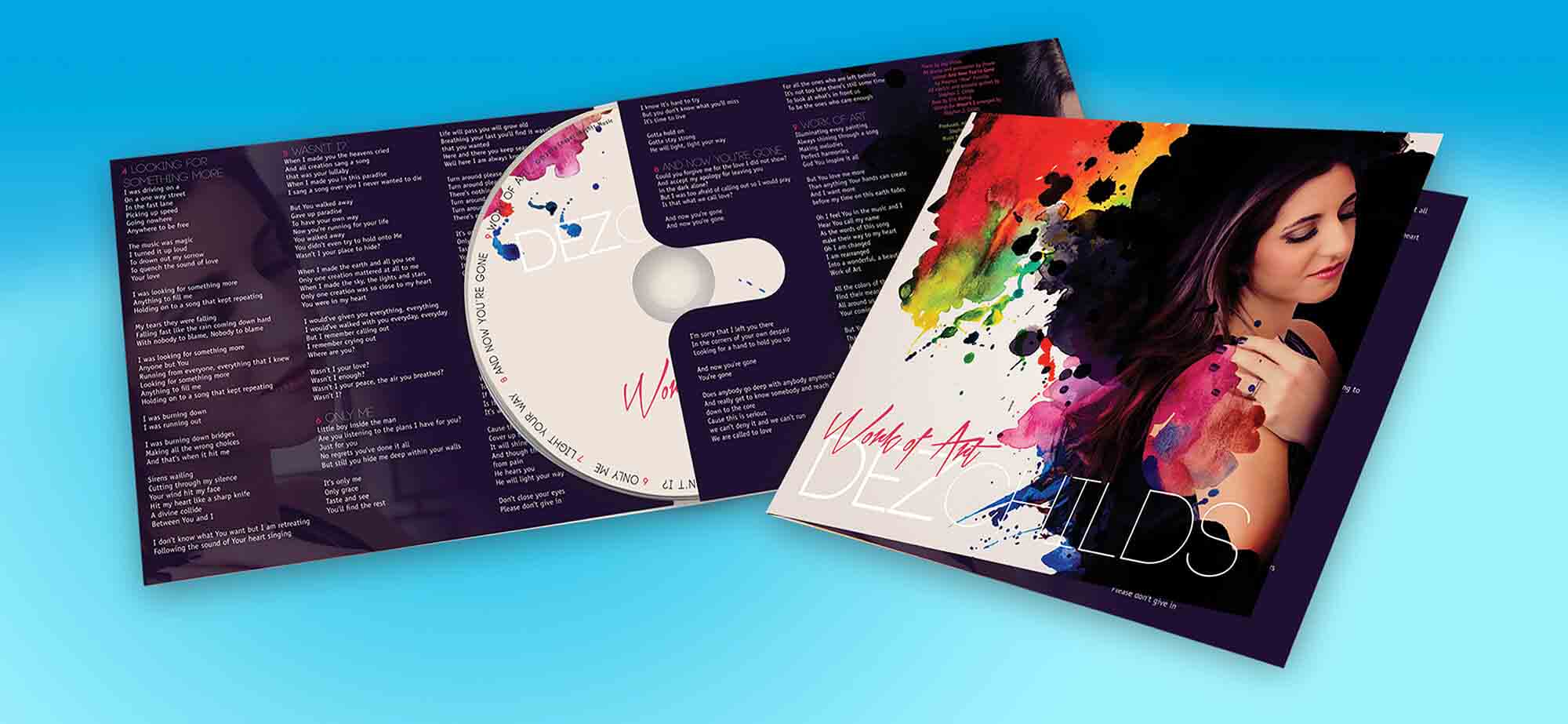The image depicts a partially open CD case with the CD itself halfway out. The CD, which has a white surface featuring colorful splotches of red, yellow, green, and orange, reads "Work of Art" in stylized cursive and "Des Childs" at the bottom. The left side of the image shows the CD booklet spread open, revealing track titles and lyrics. The right side of the image highlights the CD cover, presenting a young woman with long dark hair dressed in a black sleeveless dress. The woman, presumed to be Des Childs, has one hand up on her shoulder. The cover’s background mixes vibrant colors of paint, echoing the "Work of Art" theme. The overall background of the image is a bright blue.